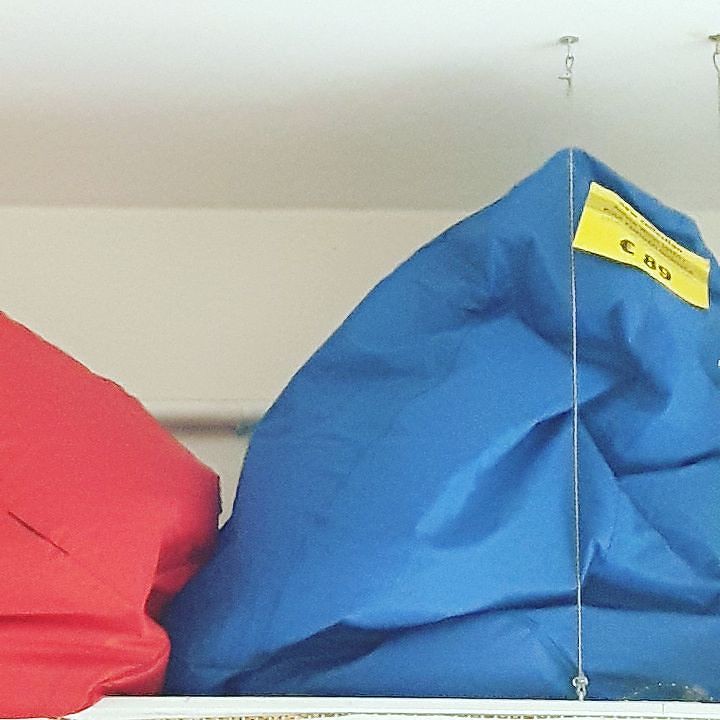In a brightly-lit room with white walls and ceiling, two vinyl bags are placed on a white shelf. The bag on the right is blue and features a yellow tag with the label "C89" written in black. Above it, additional unreadable text is present. The red bag on the left appears partially cut off in the photo but is made of similar material. Both bags are secured on the shelf by a string extending from the ceiling. The room's minimalistic design includes a light source that illuminates the scene, although the fixture itself is not visible in the photograph.